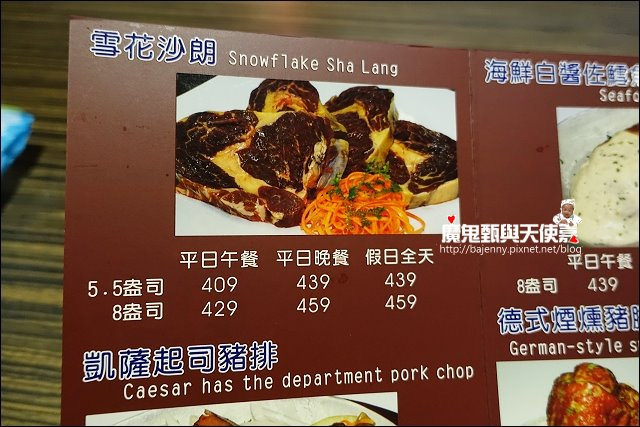The image features a Chinese menu prominently displaying a dish called "Snowflake Shaoling," which consists of raw steaks accompanied by spicy condiments. The menu includes various items written in Chinese characters, making it challenging to decipher for non-Chinese speakers. Below the Chinese text, there is an item labeled "Chinese Caesar," which intriguingly includes a "department pork chop." Additionally, a portion of the menu mentions a German-style dish, though the details are partially obscured in the corner of the image. The prices are listed in yen, with options ranging from 409 to 459 yen, likely depending on the portion size. The menu is laid out on a standard table, and someone appears to be examining it. The image primarily highlights the Snowflake Shaoling dish amidst an array of other intriguing offerings.